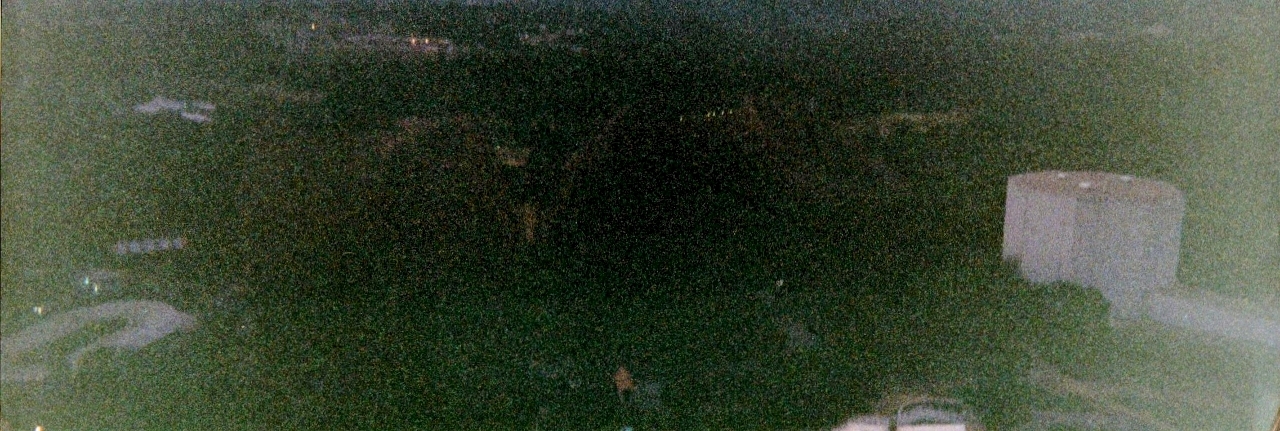A grainy, out-of-focus photograph, likely taken with a 35mm camera. The outdoor scene appears to have been captured from a high vantage point, possibly a cliff. On the right side of the image, a white domed building, approximately four stories tall, stands prominently. The background is predominantly dark, with patches of green suggesting the presence of woods or dense foliage. In the distance, more structures are faintly visible—white buildings that seem to be illuminated. Additional white buildings with lights can also be seen in the lower left corner of the image.